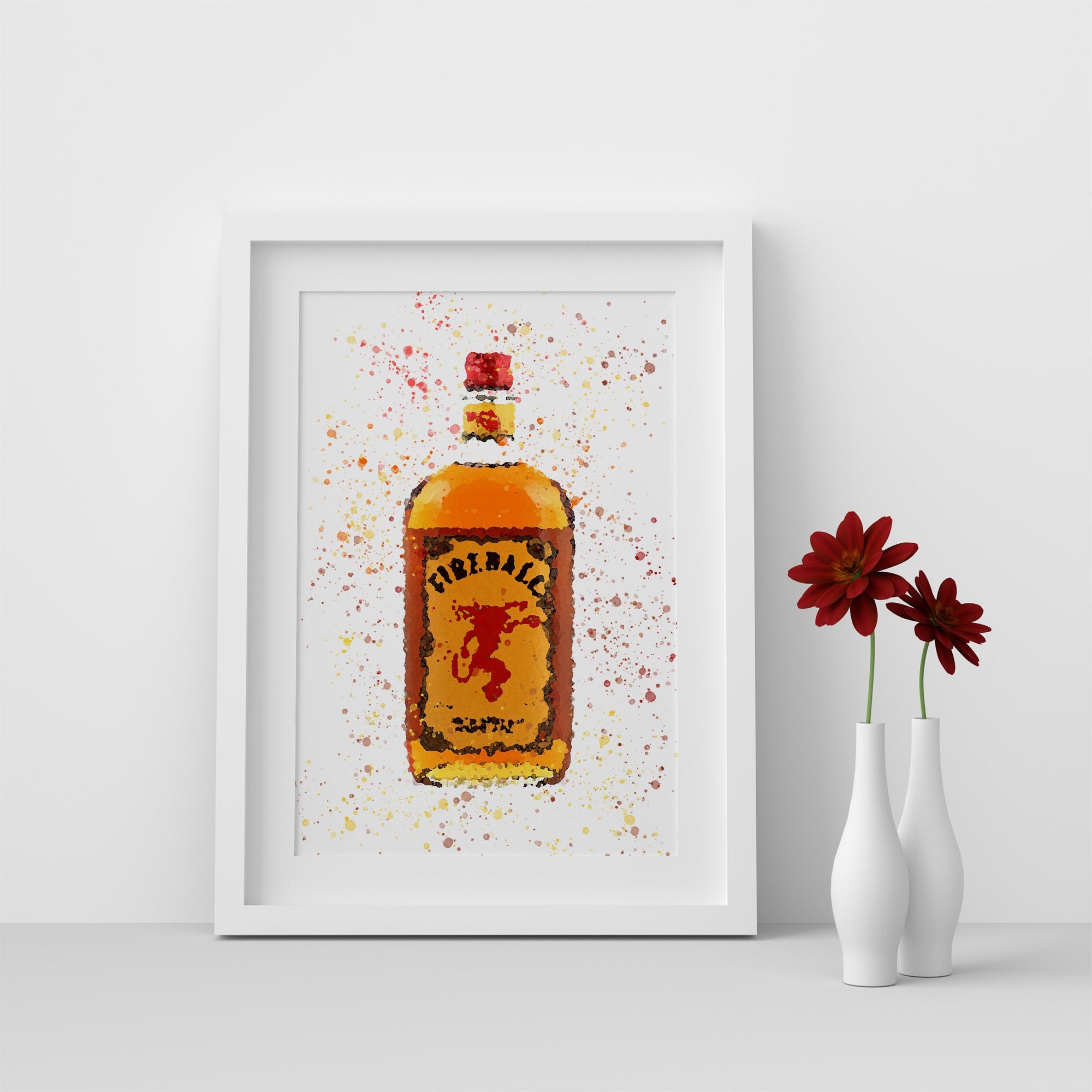The photograph showcases a minimalist setting consisting of a white table and a white wall. Central to the composition are two slim white vases, each containing a single red flower on a slender stem. Dominating the scene is a white-framed illustration with white matting, set against a white background splattered with muted red and gold tones. This stylized artwork prominently features a bottle of Fireball whiskey. The bottle, filled with amber-colored liquid, has a worn-looking label. The label, set on a yellow background, displays the word "Fireball" in black letters, accompanied by a red, devilish creature reminiscent of an upright goat or possibly a lion. The bottle is capped with a red top. The overall aesthetic of the image is clean and modern, with a monochromatic palette accented by vibrant reds.